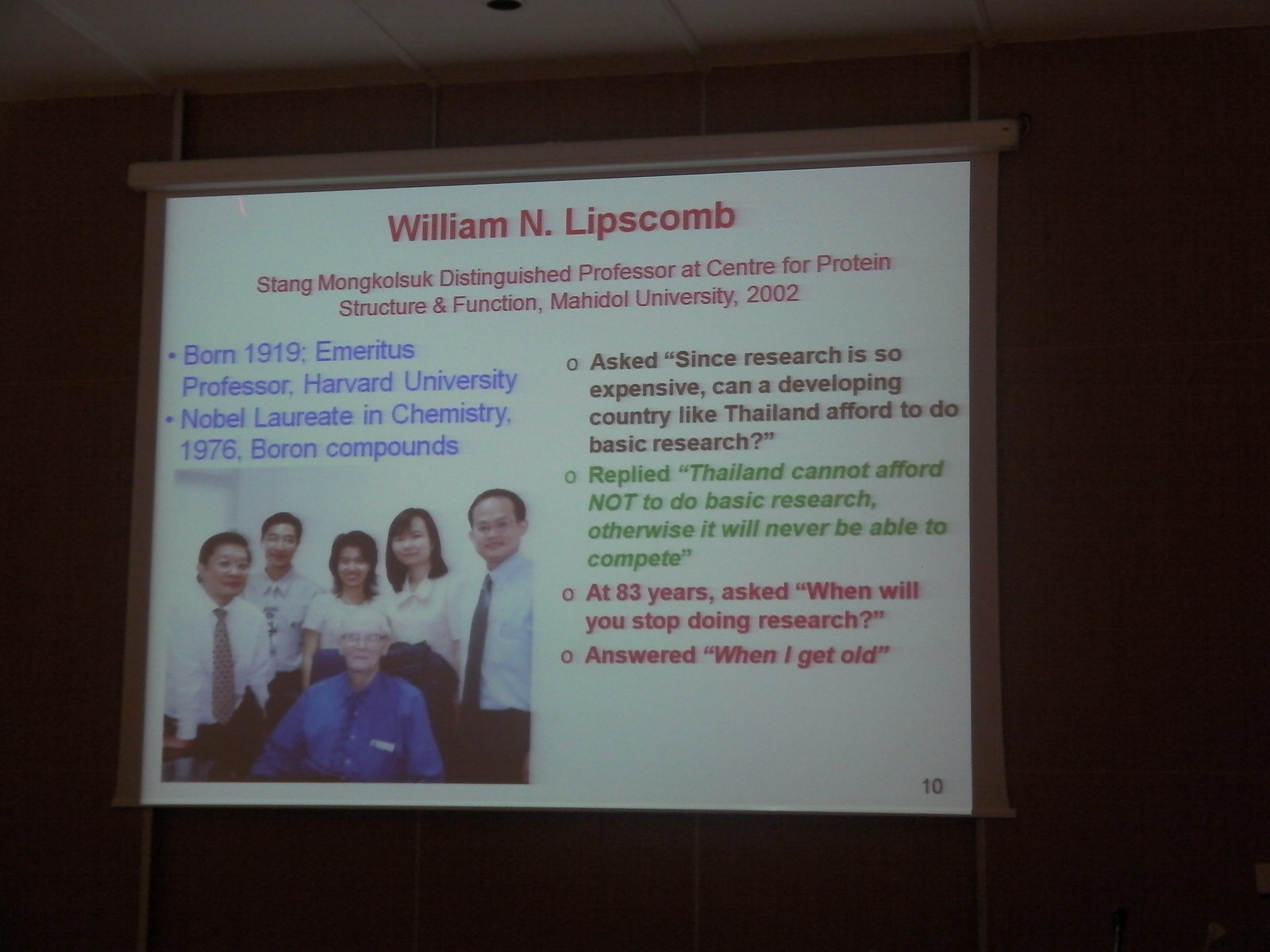This is a detailed photograph of a projected presentation slide paying tribute to William N. Lipscomb. The slide features text detailing his illustrious career, stating that he was the Stang Mongkolsuk Distinguished Professor at the Center for Protein Structure and Function at Mahidol University in 2002. Born in 1919 and an emeritus professor at Harvard University, Lipscomb was a Nobel Laureate in Chemistry in 1976 for his research on boron compounds. The presentation also highlights a notable Q&A session where Lipscomb was asked whether developing countries like Thailand can afford to do basic research. He emphatically replied, "Thailand cannot afford not to do basic research; otherwise, it will never be able to compete." At 83 years old, when questioned about retiring, he humorously answered, "When I get old." The slide includes a picture of Lipscomb wearing a blue button-up shirt, sitting surrounded by five colleagues in white shirts. The text is color-coded with significant portions in red, blue, brown, and green to emphasize different sections and questions.